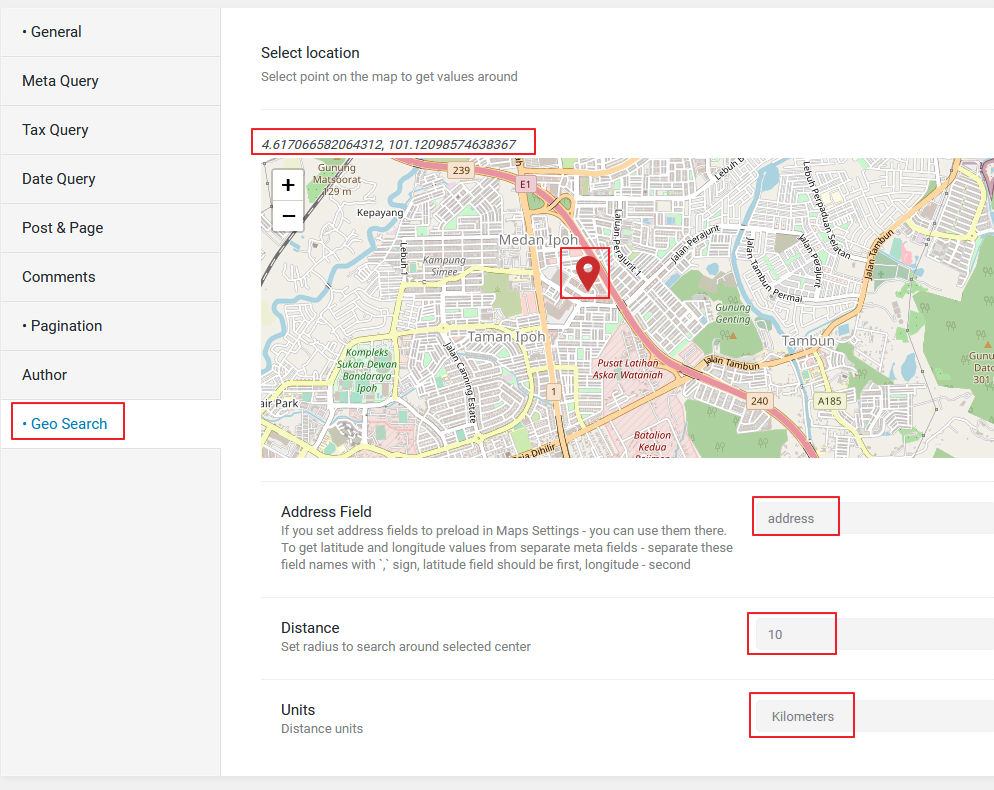Certainly! Here is the polished and detailed caption for the image:

---

The image displays a webpage interface. On the left side, there is a vertical gray menu listing the following options: "General," "Meta Query," "Tax Query," "Data Query," "Post and Page," "Comments," "Pagination," "Author," and "GeoSearch." The "GeoSearch" option stands out with a white background and blue text, encased in a red border.

To the right of the menu, the main content area appears on a white background. At the top, the title "Select Location" is prominently displayed in bold black text. Below this, an instructional message in gray font reads, "Select point on the map to get values around." 

A red-bordered numeric string, "4.617066582064312, 101.12098574638367," is visible, likely representing geographic coordinates. Directly below, a map is shown, complete with zoom controls (a plus and minus sign) and labeled streets and points of interest.

Further down, sections labeled "Address Field," "Distance," and "Units" are present, each accompanied by open fields where users can input data pertaining to addresses and distances.

---

This revised caption provides a clear and comprehensive description of the webpage displayed in the image, covering all visual elements and their respective functions.